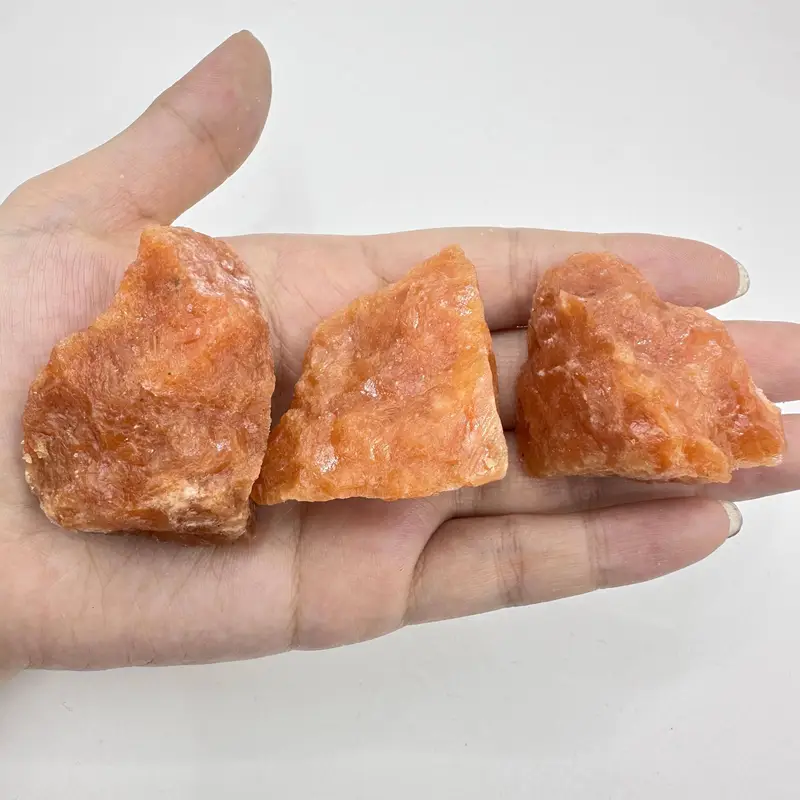A detailed close-up image captures a light-skinned left hand, outstretched and holding three orange-yellow rocks of varying shapes and sizes. Each rock appears to have a jagged, almost quartz or granite-like texture, with their hue shifting from dark burnt orange at the base to lighter, nearly white streaks at the tops. The fingers, with long, untrimmed fingernails, cradle the rocks in a way that spans from the palm to the tips, suggesting somewhat large, hand-sized stones. The hand is oriented sideways, with the thumb at the top left and the fingers extending to the right. The background is a stark white, emphasizing the intricate details and color variations of the rocks.